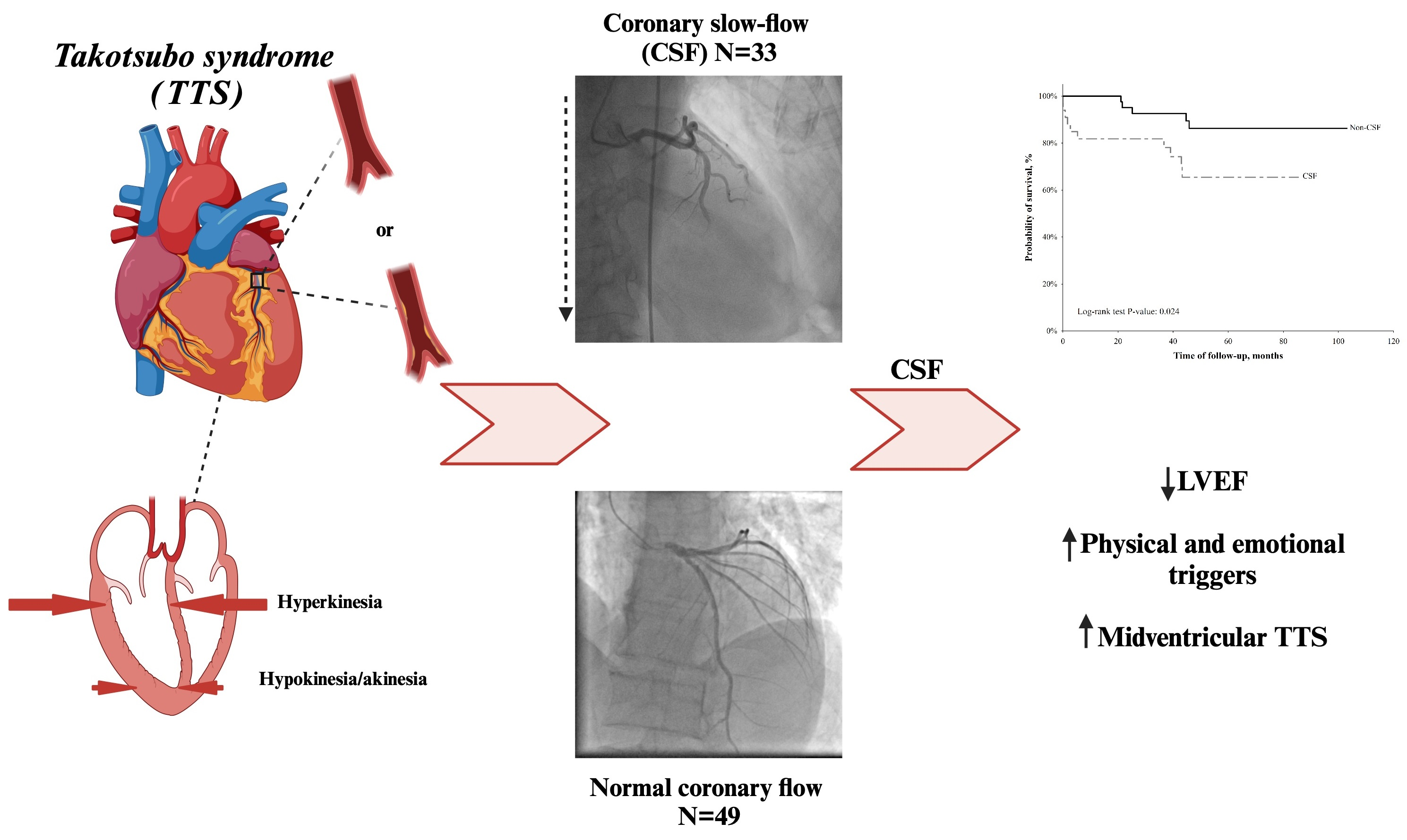The image is a detailed medical diagram focusing on Takotsubo Syndrome (TTS). In the upper left corner, the title "Takotsubo Syndrome (TTS)" is prominently displayed next to an illustration of a heart. Below this, a cross-sectional diagram of the heart features detailed annotations. Arrows point to parts of the heart labeled "hyperkinesia" and "hypokinesia/akinesia."

In the center of the diagram, there are two comparative images, likely x-rays, showing different coronary flows. The first image, labeled "coronary slow flow (CSF), n=33," illustrates restricted blood movement through a major heart vessel. The second image, labeled "normal coronary flow, n=49," shows typical blood flow through the vessels. Red arrows and additional labels clarify that "CSF" stands for coronary slow flow.

To the right, the diagram features a graph detailing coronary flow variations and includes notations such as "LVEF" (Left Ventricular Ejection Fraction) with a downward arrow, indicating a decrease, and upward arrows annotating "physical and emotional triggers" and "midventricular TTS." Additional text and smaller arrows further explain the significance of these factors, providing a comprehensive overview of the syndrome and its impact on heart function.